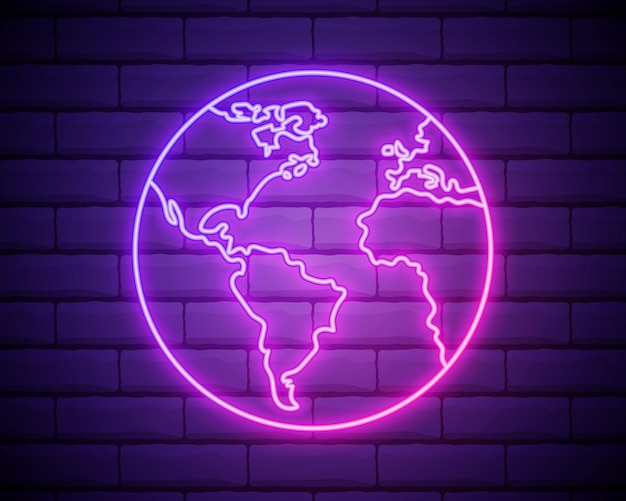The image features a neon sign depicting a globe, mounted on a textured brick wall. The bricks exhibit various shades of blue and purple, giving the background a multi-tonal appearance, with darker sections in the corners where the lighting is less intense. The glow from the neon sign accentuates these shades, adding to the visual complexity. The globe itself is outlined in thin, white neon lines, with a bright pink circumference encasing it. Within the globe, North and South America are prominently visible to the left, while parts of Africa and a slightly obscured Europe, including a distinct Italy, can be seen on the right. The neon lights cast a purplish and pinkish hue across the wall, further enhancing the mystique of the image, making it difficult to distinguish whether it is a realistic photograph or a rendering.